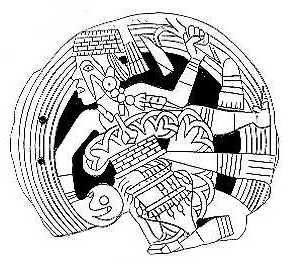This intricate black and white illustration, potentially hand-drawn or digitally rendered, portrays a figure steeped in ancient and modern elements. The figure is depicted as a deity-like man, skewed at a 45-degree angle to the left, encapsulated within a partially complete circle with parallel lines radiating outward, creating a dynamic frame. The man, adorned in what appears to be a traditional and ornate costume, wears a substantial flat-topped headdress adorned with feathers and beads cascading from his eyes, evoking an Egyptian motif. His left hand clasps a globe-like object, while his right hand holds a plant or weapon-like item. Further adding to the figure's elaborate attire, he sports large, circular earrings. The background within the circle is pitch black, suggesting a cosmic or otherworldly setting, enhancing the illustration's mystique. The figure appears almost brick-like with its many squares, giving it a textured, multifaceted appearance as it hovers seemingly weightless in this abstract universe.